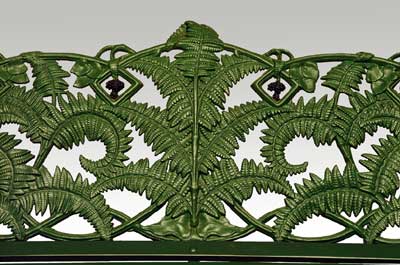The photo displays an ornate, decorative metal piece, likely a topper for a fancy metal gate or archway. This metal design is painted green and prominently features symmetrical, intricate scrollwork centered around fern leaves. Down the middle, a central green stem supports three sets of paired fern leaves, arranged in rows with each pair curving outward to the left and right. At the top, the structure is crowned by an arch flanked by two small triangles containing intricate designs. Complementing the central column, similar fern patterns and curls extend to the sides, adding to the elaborate artistry. The background is gray, providing a contrast that highlights the green of the metal, and a thick, dark green, straight, and flat metal bar stretches across the bottom of the piece, anchoring the intricate design.